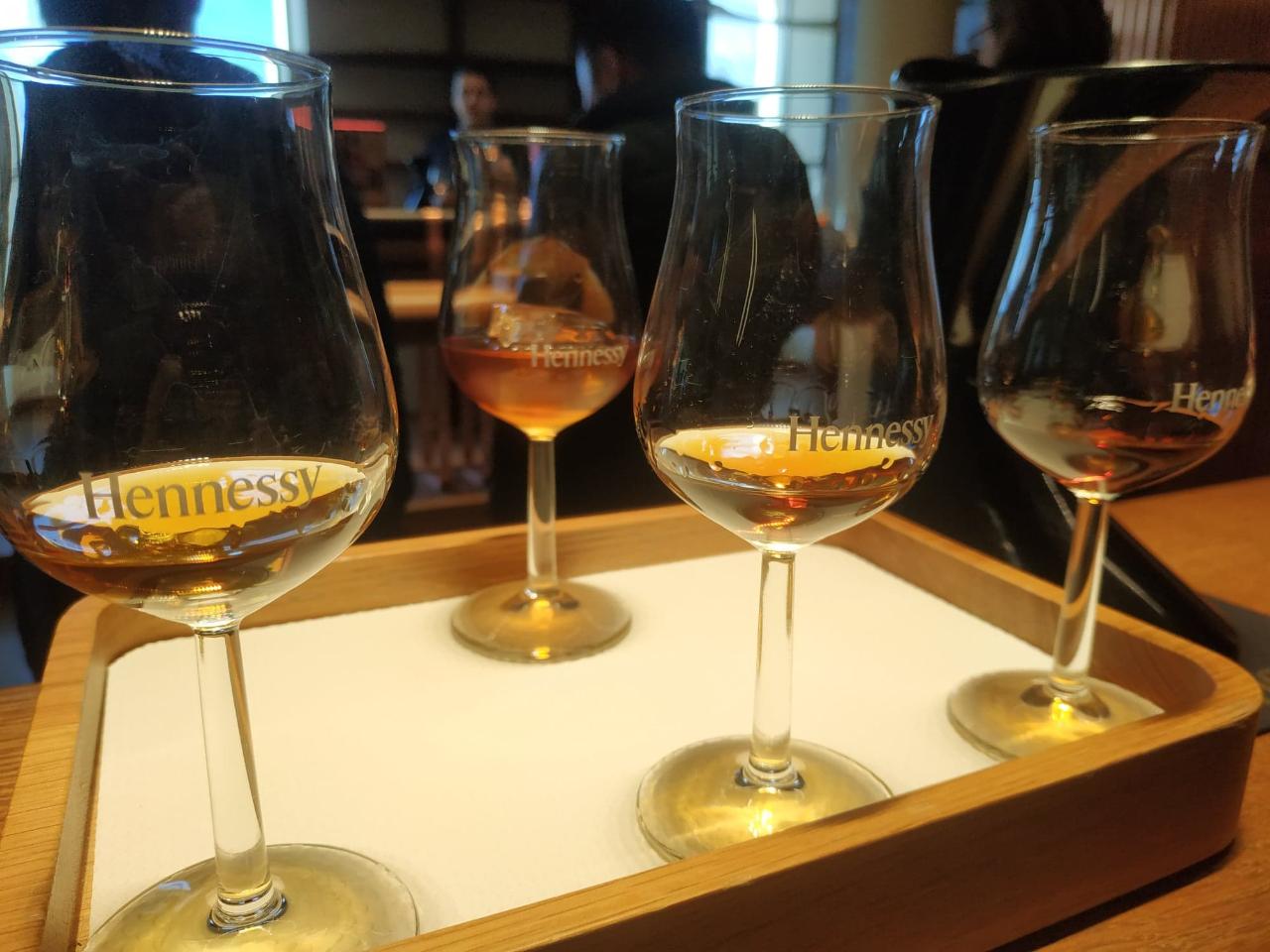This realistic photograph, oriented horizontally, captures a close-up scene inside a slightly darkened restaurant or bar. In the background, there are beige walls and dual windows framing a dimly lit area where a few people are seated. The foreground focuses on a light brown wooden table, atop which rests a meticulously detailed serving tray. The tray features a white, square bottom with rounded edges and light brown wooden rails elevated about an inch above the base. 

On the tray are four elegant whiskey snifters, each with a round base, a two- to three-inch tall stem, and a bulbous, rounded cup designed for sipping whiskey. The glasses, uniformly labeled with "Hennessy" in white font, are approximately a fourth full with a brownish-amber liquid, presumably Hennessy whiskey. The composition, with its emphasis on the drinkware and the subtle background details, draws attention to the refined presentation of the whiskey and the understated ambiance of the establishment.